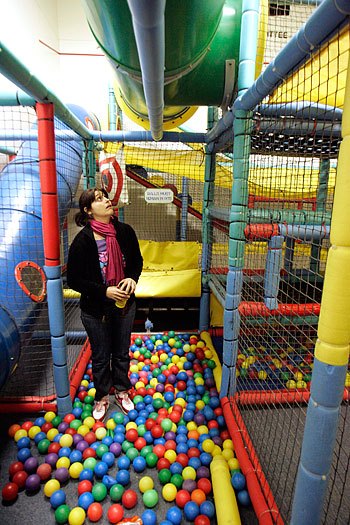The image captures a vibrant children's play area dominated by a colorful ball pit filled with an assortment of red, yellow, green, and blue plastic balls. The ball pit is enclosed by netted screens and foam pillars in shades of red, green, and blue, forming a maze-like structure. Overhead, a large green plastic tube and various slides, including a blue slide on the left and a yellow slide in the background, add to the playful environment. At the center, a woman stands in the ball pit, gazing up at the structure. She is dressed in a black long-sleeve shirt with purple showing underneath, black jeans, and white and red shoes. Her outfit is accentuated by a red scarf and long, tied-back brown hair. She holds a white or yellow cup in her hands and has a pink scarf around her neck. The mixed colors of the play area also include gray, with netted cages, segments for climbing, and crawl pipes completing the engaging setting.